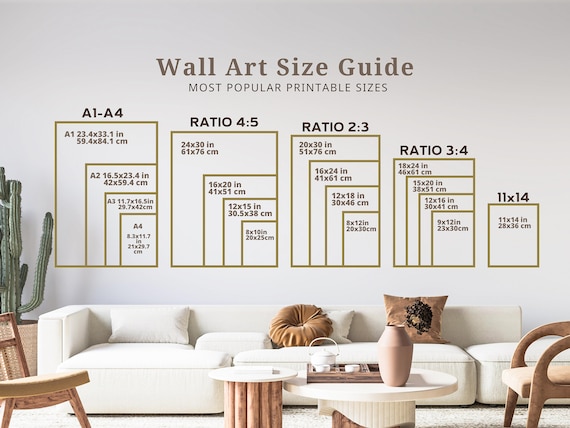This detailed photograph showcases a modern, minimalist living room with a white sofa against a gray wall, adorned with brown pillows. To the left of the sofa stands a three to four-foot tall cactus, adding a touch of greenery to the space. In front of the sofa, two small coffee tables contribute to the contemporary décor. The room serves as a backdrop for a "Wall Art Size Guide," displaying the most popular printable sizes. Overlaid on the wall are various rectangles, each containing smaller rectangles that represent different print sizes such as A1 to A4, 4:5 ratio, 2:3 ratio, 3:4 ratio, and 11x14 frames. These visual aids help viewers gauge the proportions and placement of wall art in a real living room setting.